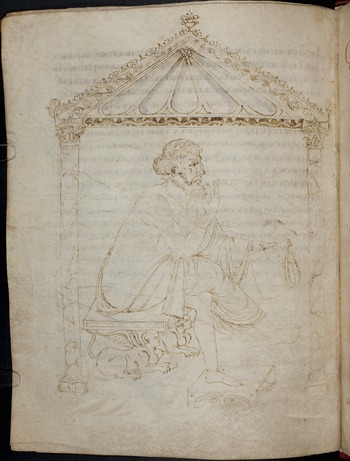The image appears to be a detailed pencil drawing, reminiscent of an ancient book illustration, potentially in the style of da Vinci. It depicts a man with long hair and a beard, possibly symbolic of a biblical figure such as Jesus, seated in a Greco-Roman style gazebo with open sides. The man is draped in a toga-like garment, suggestive of Greek or Roman attire, and sits on a bench supported by two peculiar creatures. These creatures are a blend of mythological elements, resembling griffins with small baby faces, prominent breasts, tiny wings, and lion-like tails and paws. The gazebo itself features intricately designed Corinthian columns supporting a highly decorated roof, possibly with art deco elements. The setting includes another figure at the seated man's feet, whose gender and age are unclear but appears to be seeking help or solace. The entire scene seems printed on a page that has indistinguishable text in the background, suggesting either an overlaid artist’s sketch on a book page or an integrated art piece within the book. The atmosphere of the image is both classical and contemplative, capturing a moment of profound empathy and thoughtfulness.